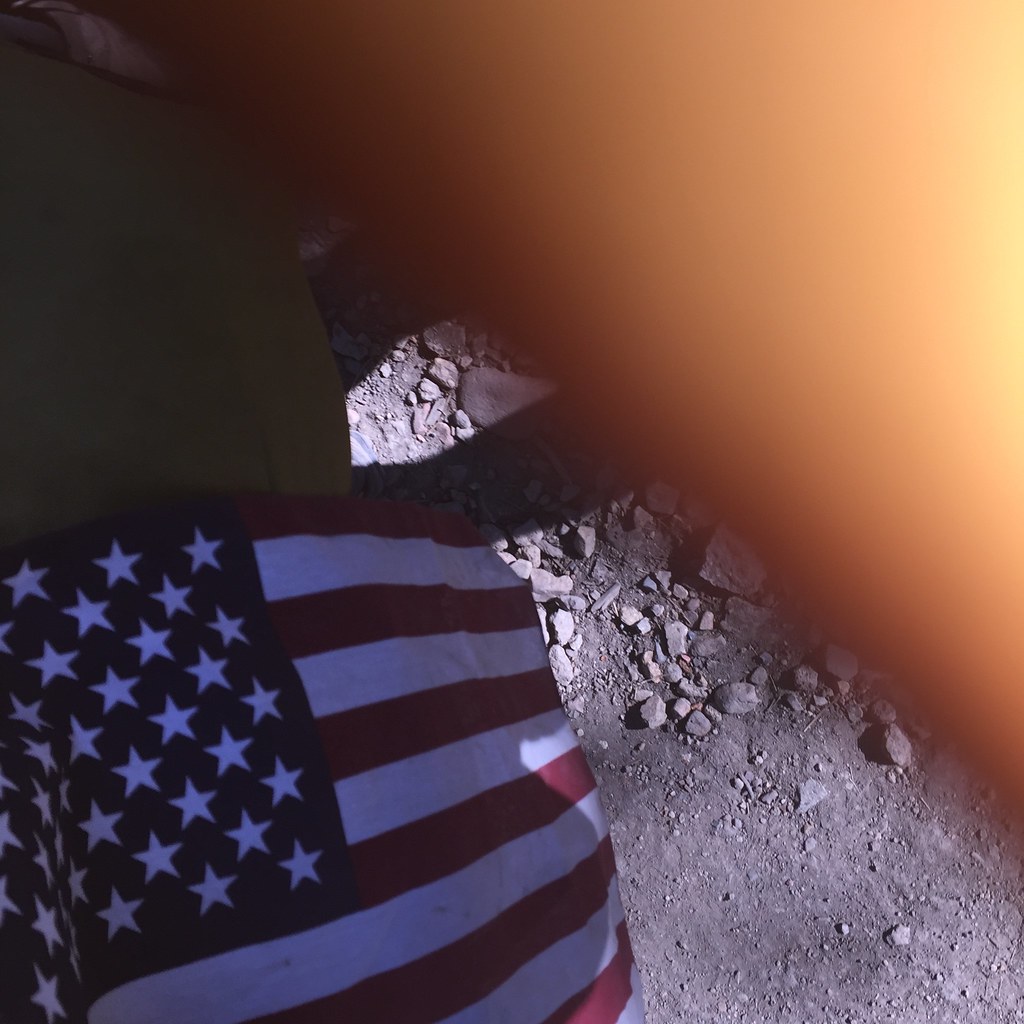A top-down view of what appears to be a lunar landscape. The image is predominantly dominated by an orange glow emanating from the top left corner, casting an orangey-yellow hue across a significant portion of the scene and gradually darkening as it spreads outward. The surface below looks like a rocky, solid ground, typical of what one might expect on the moon. On the bottom left of the image, the American flag is prominently displayed, featuring white and red stripes with a blue square in the top left corner containing 50 white stars.